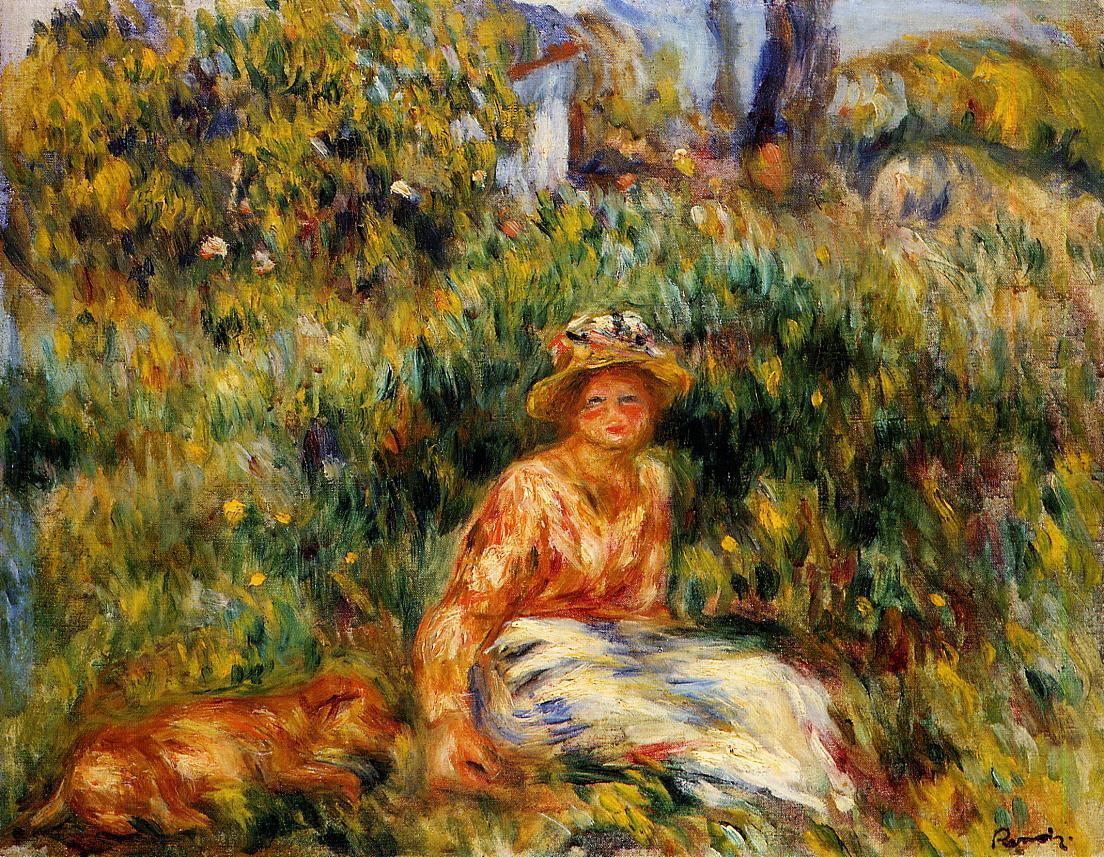This is an Impressionist oil painting titled "Young Woman in a Garden" by Pierre-Auguste Renoir, created in the late 1800s. The scene is set in a field abundant with flowers, indicative of a vibrant spring day. At the center of the image, a young woman is depicted lounging on the grass. She wears a white skirt and an orange shirt, topped with a sun hat adorned with flowers. The broad, sketchy paint strokes that form her face and body give the painting a textured, canvas-like appearance. By her side lies a brown dog, seemingly at peace. The background features an array of trees, bushes, and greenery, with a hint of blue sky and distant hills. An artist’s signature is seen in the bottom right corner, and the composition is presented in a landscape orientation.